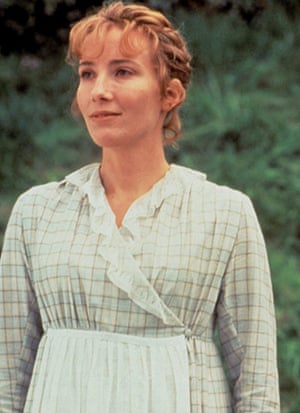This photograph features a fair-skinned woman with reddish-brown hair styled in an updo and curly bangs. She is shown from the head to part of the torso, standing with her arms at her sides. The woman's slight smile and gaze directed into the distance to the left convey a sense of contemplation. She is adorned in an older style dress, which features a plaid checkered pattern in pale cream and white colors, and possibly blue, with a grid running through it. The dress is accessorized with white lacy furrows down the front and a ruffly white collar, giving it a traditional and somewhat old-fashioned appearance, with an apron that could be part of the dress. The photograph is set outdoors during the daytime against a backdrop of green foliage, likely bushes, adding a natural, serene atmosphere to the image.